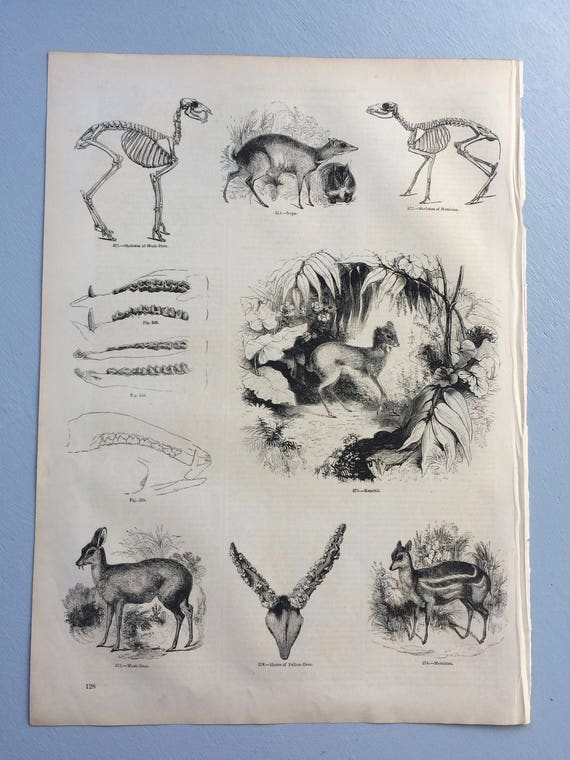This is an image of page 128 from an old, worn book, showcasing a variety of black-and-white illustrations of deer-like creatures and skeletal structures. The page has eight drawings arranged with three small illustrations at the top, two larger ones in the middle, and three more small drawings at the bottom. Among these, there are intricate depictions of deer species, both modern and prehistoric, including two skeletal deer and imaginative hybrids. One illustration stands out with a floral wreath surrounding the deer, possibly a nod to a nature-themed representation. Additionally, the page features detailed diagrams of dental patterns and skull structures, including a prominent front-facing skull with V-shaped horns. The page also has a jagged right edge, indicating it was torn from its binding. This eclectic collection offers a window into the diversity of the cervid family and related species.